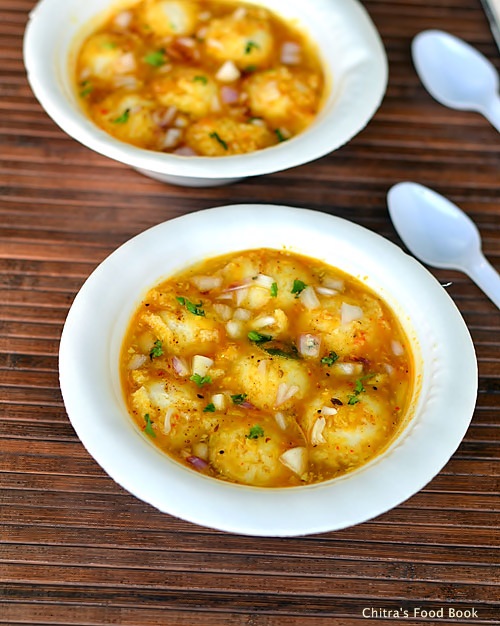In this appetizing image, captured on a light brown wooden table with a rich, grainy texture, the lower right corner features the text "Chitra's Food Book" in crisp white letters. Central to the presentation are two large white bowls, brimming with plump Chinese dumplings, delicately garnished with finely chopped onions and chives. The dumplings are generously drizzled with a savory brown sauce, which adds a tempting sheen to the dish. Flanking the bowls on the table, two humble plastic spoons attest to the casual, yet inviting, nature of this culinary scene. The overall composition exudes warmth and flavor, making the bowls of dumplings appear irresistibly delicious.